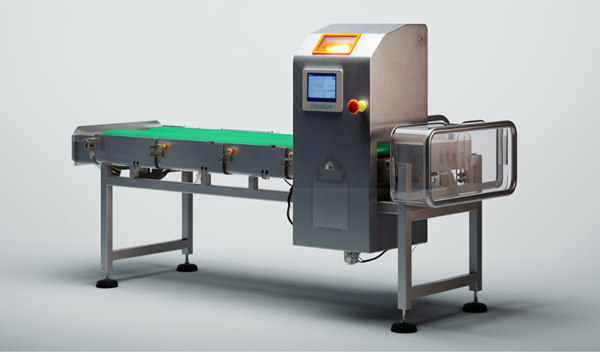This photograph captures a sophisticated piece of machinery, possibly used in a medical or security setting. The machine has a rectangular, metal body with four legs, each ending in suction cup-like feet, lending it stability. Dominating the structure, there is a green conveyor belt that protrudes from one side, likely for scanning or transporting items. 

On its front, a detailed array of components includes a red push button and a small screen, complemented by a gauge situated below another gauge encased in a yellow frame on top of the machine, indicating it might monitor different parameters. A clear, suitcase-shaped box, possibly for storing or inspecting contents, is visible at one end. The machine is intricately connected with various wires, suggesting complex electrical or signal processing capabilities. Silver sides and a green blanket-like covering resemble features of a table or bed, further hinting at its versatile application in both medical and industrial environments.